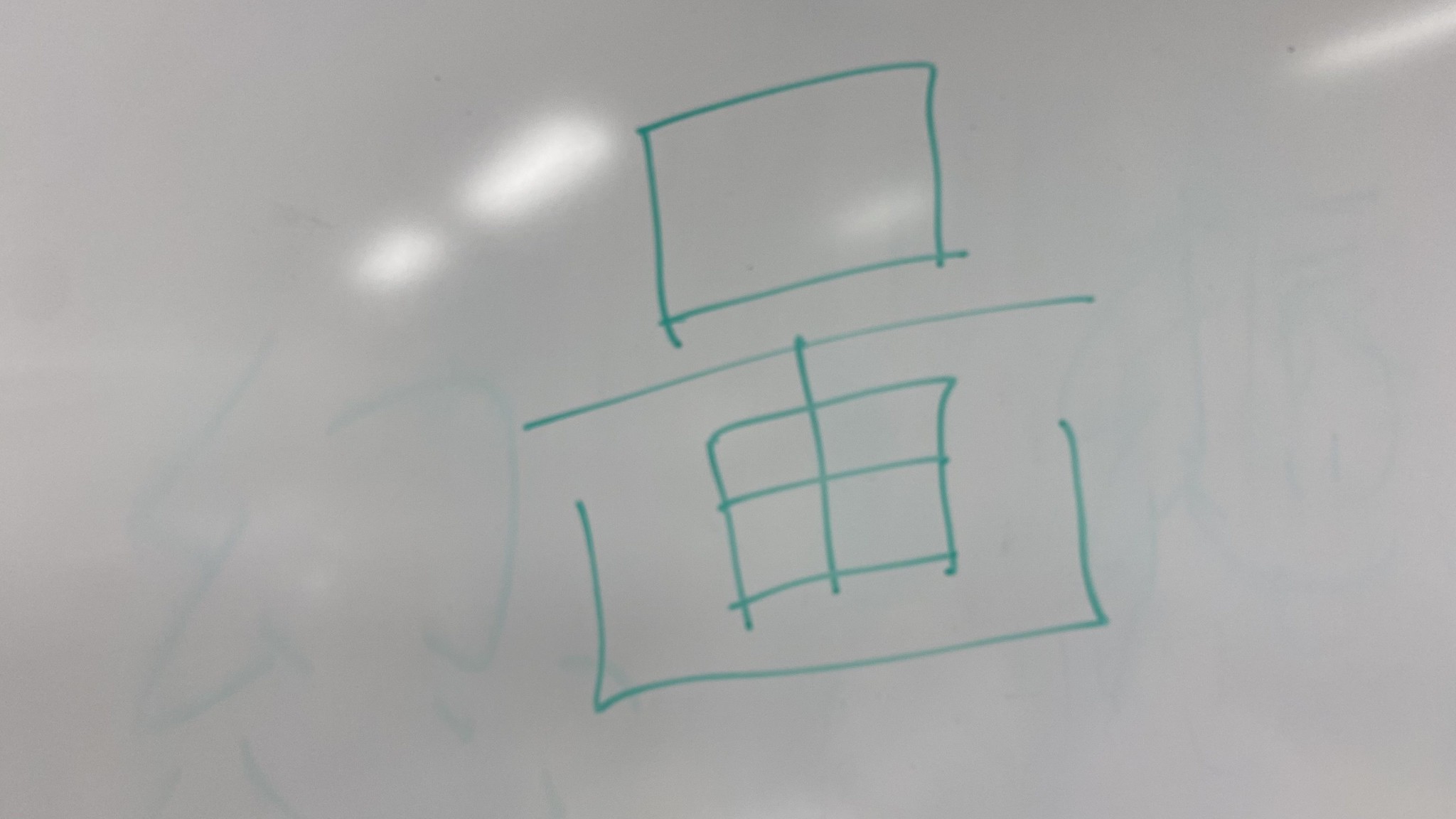This is an image of a whiteboard drawing, created with what appears to be green marker. At the top center of the whiteboard, slightly tilted to the left, there is a large square. Below this square, a horizontal line extends beyond the square’s edges, and from its center, a vertical line descends, forming a large T-shape. Underneath this T-shape, there is another square, resembling a window, divided into four smaller squares. Beneath this window-like square, there is a straight horizontal line with two vertical lines rising from its ends, forming a U-like shape. To the left of these drawings, remnants of a bell shape are faintly visible, suggesting it has been partially erased. Additionally, in the middle section of the whiteboard, there are reflections of oval-shaped ceiling lights from the room, adding a subtle reflective quality to the image.